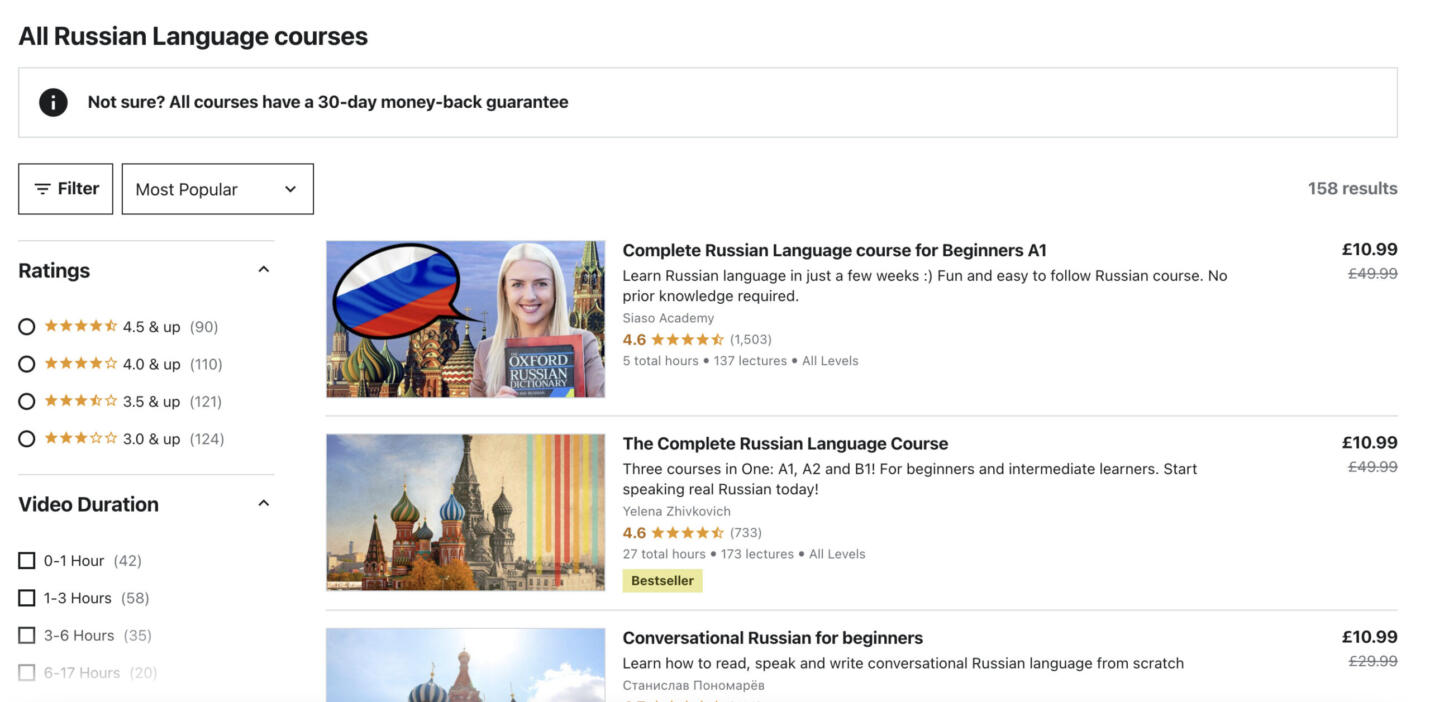This image captures a section of a webpage dedicated to Russian language courses. At the top of the page, a header reads "All Russian Language Courses" followed by a reassurance that "Not Sure? All Courses Have a 30-Day Money-Back Guarantee." Below this, there is a filter section allowing users to sort courses by popularity and ratings, with options to select ratings of 4.5 stars and higher, 4 stars and higher, 3.5 stars and higher, or 3 stars and higher. The duration of courses can also be filtered, with selectable time ranges including 0 to 1 hour, 1 to 3 hours, 3 to 6 hours, and 6 to 17 hours, although the remainder of the choices is cut off in the image.

In the upper portion of the visible courses, there is a class titled "Complete Russian Language Course for Beginners A1," which is rated 4.6 stars, depicted in yellow. This course offers a total of 137 lectures spanning 5 hours and is suitable for all levels. The price of this course is listed as £10.99. 

Below this, another course is listed: "The Complete Russian Language Course," which is described as offering three courses in one. This course also holds a rating of 4.6 stars, is marked as their best seller, and has the same price of £10.99. The image cuts off partway through the listing of a third course at the bottom.